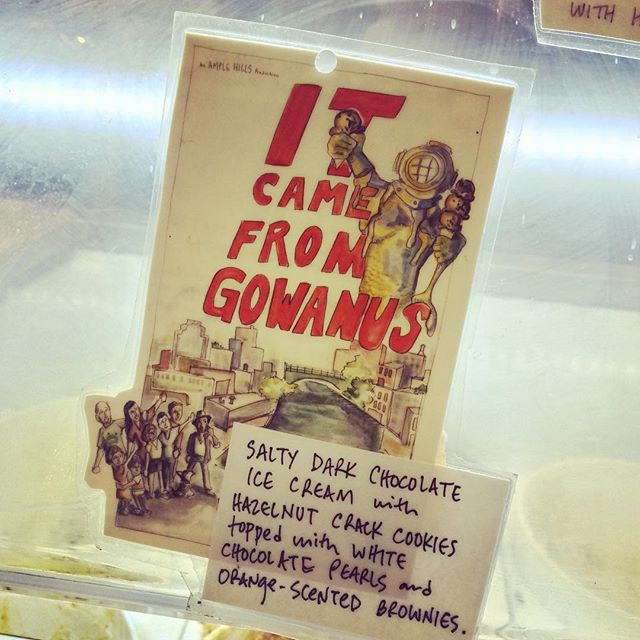The image displays a creatively designed sign taped to a transparent display case covering several tubs of ice cream. Dominating the sign is a comic book-style illustration featuring a swimmer or diver equipped with an old-fashioned scuba diving helmet, towering above a cityscape with a canal and bridge. The diver-monster character holds an ice cream cone in each gloved hand—the one in the right holds a single scoop, while the left cone boasts three scoops. Surrounding the monstrous figure are tiny people at the bottom, looking up and pointing at the spectacle with a mix of awe and amusement. The sign dramatically declares in bold red text, "It came from Gowanus," capturing attention with its vibrant lettering. Additionally, a secondary sign attached to the dome lists the flavor details: "Salty dark chocolate ice cream with hazelnut crack cookies topped with white chocolate pearls and orange scented brownies." This elaborate label, unlike the more subdued labels of other flavors seen at the bottom left and right, adds a touch of whimsy and charm to an already delightful scene.